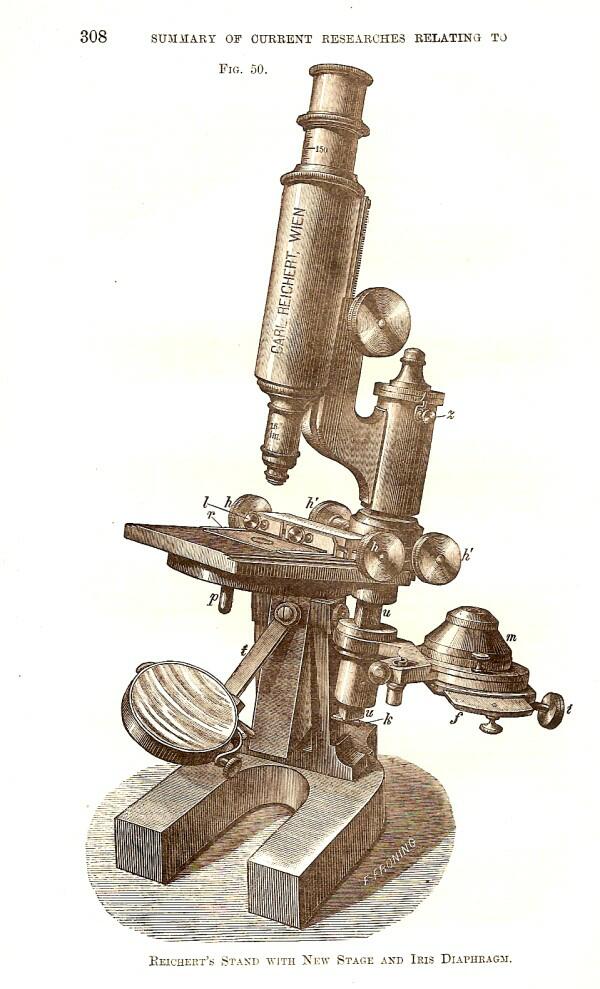This hand-drawn illustration of a microscope appears to be a detailed schematic, possibly from an 18th or 19th-century science book or encyclopedia. The image features a vintage-looking microscope labeled with "Carl Reichert, Wien" at the top, suggesting its Austrian origin. The top-left corner prominently displays the numbers "308" and "Figure 50," while a heading above reads, "Summary of Current Researches Relating to." The diagram meticulously depicts various parts of the microscope, including different lenses and attachments, and is annotated with letters H, Z, P, T, K, U, M, and F, whose explanations are presumably on a facing page. The base of the illustration notes, "Reichert's stand with new stage and iris diaphragm," highlighting its advanced optical features. The color scheme is predominantly brown and goldish-copper, adding to its antique appearance.